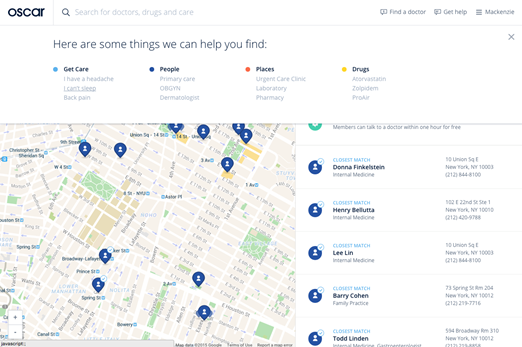This is an image of a website map interface from a platform named "Oscar," displayed in lowercase dark blue text. The interface prominently features a search bar with the placeholder text "search for doctors, drugs, and care," accompanied by a search icon. 

To the right, there are several navigation options: "find a doctor," "get help," and a user profile labeled "McKenzie." 

Beneath these, the site offers assistance with four specific categories indicated by colored bullet points. In light blue, "Get Care" includes options like "I have a headache," "I can't sleep," and "back pain." The dark blue section, "People," lists medical professionals such as "primary care," "OBGYN," and "dermatologist." The red circled section "Places" covers facilities like "urgent care clinics," "laboratories," and "pharmacies." Lastly, the yellow circled "Drugs" section mentions specific medications, including "Atorvastatin," "Zolpidem," and "Prozac."

The left-hand side of the interface features a densely populated map with multiple dark blue location pins indicating various service providers. Adjacent to the map, on the right side, there is a list of these locations and their details. Each entry includes the name of the medical professional, their specialty, and their address. For example, the closest match displayed is "Donna Finkelstein, internal medicine, located at 10 Union Square, New York, NY 10003," with a contact number of "212-844-8100." Other listings include names like "Henry Beluda," "Lee Lin," and "Barry Cohen," all specializing in internal or family medicine. 

Overall, the interface seems to facilitate easy navigation and resource finding, albeit with the small, fuzzy font making some details challenging to read.